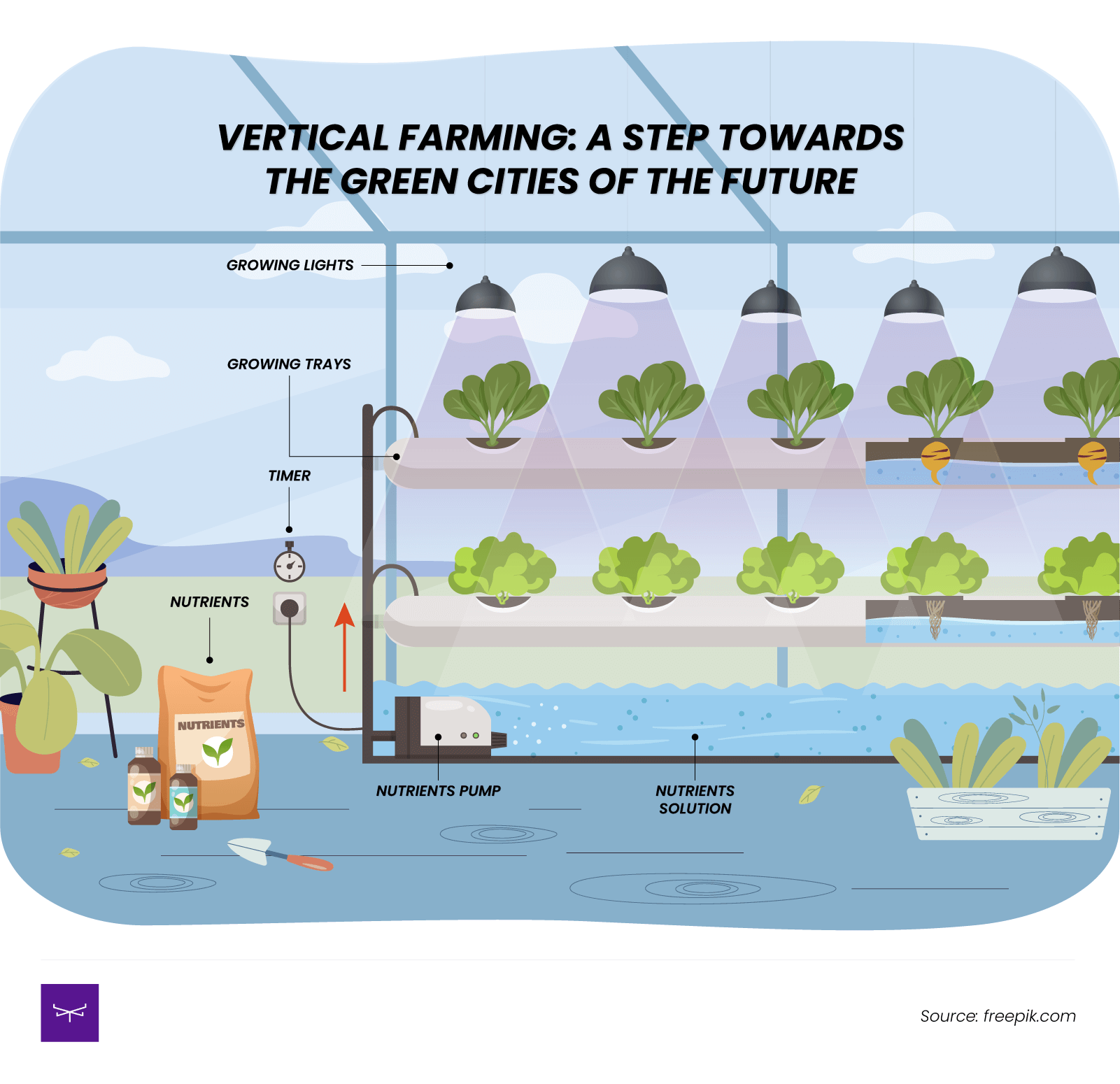The image is a detailed and colorful graphical poster made for educational purposes, focusing on vertical farming as a step towards sustainable green cities of the future. The poster features a square layout with undulating top and bottom edges, and rounded corners. The text at the top reads, "Vertical Farming: A Step Towards the Green Cities of the Future," all in black font.

The main visual depicts the interior of a greenhouse with an organized vertical farming system. In the right section of the image, there are multiple rows of green plants growing in labeled "growing trays" with dome-shaped black "growing lights" positioned above each tray to provide the necessary illumination. On the left, additional plants are shown in pots alongside a brown bag marked "nutrients" and two bottles. 

A timer is visible, labeled simply as "timer," which controls the delivery system for water and nutrients. The bottom section of the image highlights a "nutrients pump," identified as black and white, sitting in a labeled "nutrient solution." Pipes are shown distributing water and nutrients to enhance growth efficiency.

In the background, a serene landscape with sky, clouds, and a mountain range can be observed, merging seamlessly into the educational theme. At the bottom right, there is a credit line indicating the source as "freepic.com."